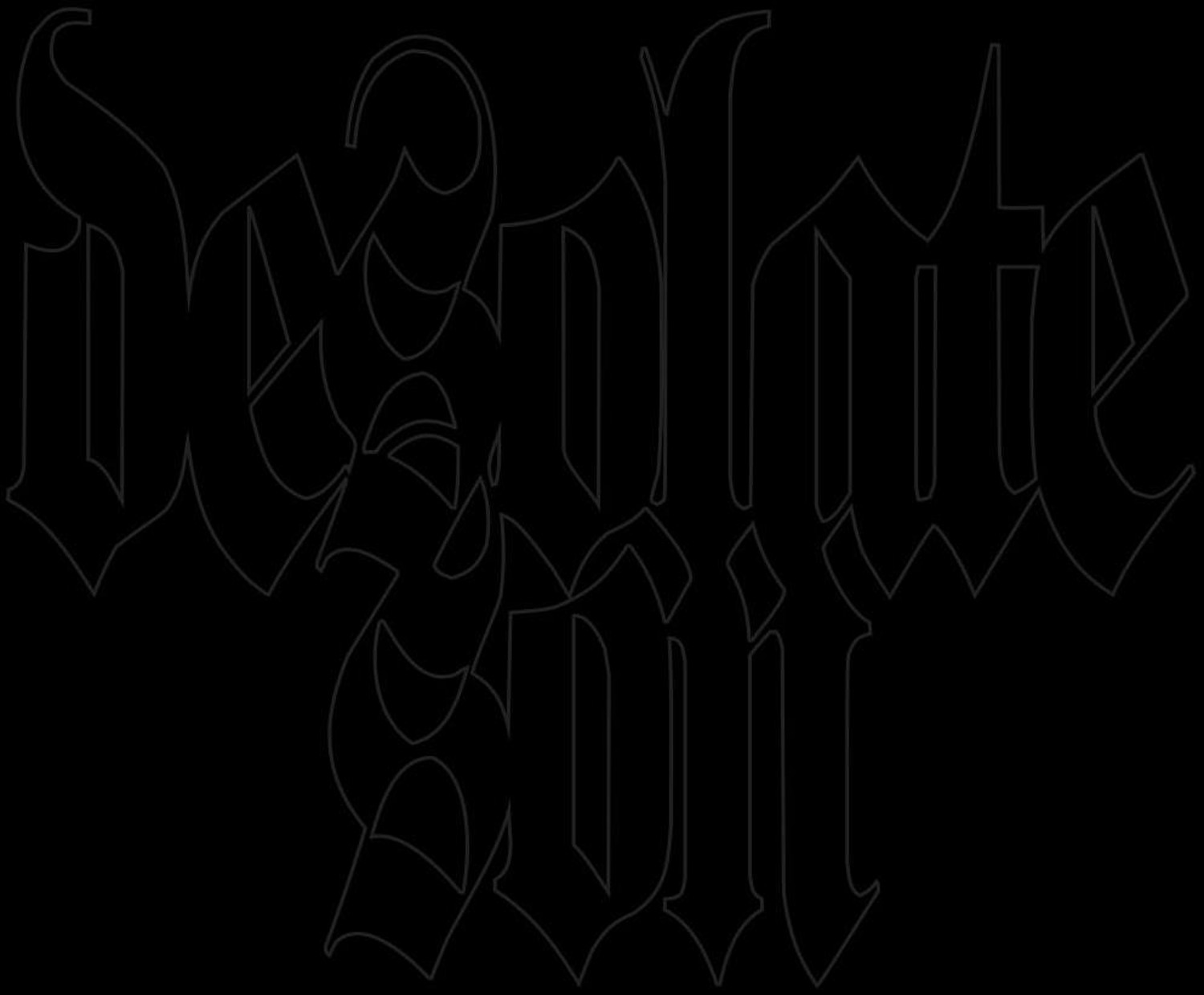The image features a completely black background with thick, decorative bubble letters that appear slightly grayish in hue. The interconnected letters, making up a single word without any gaps or separations between them, are difficult to decipher due to the dark backdrop. After close examination, it seems the word starts with "DE" and possibly spells "DESOLATE," with some interpretations suggesting additions like "SOIL." The stylized, compact design of the letters, all touching and seamlessly connected, adds to the challenge of reading the text, suggesting the creative intention behind the text might be a band name or a logo with an environmental theme.